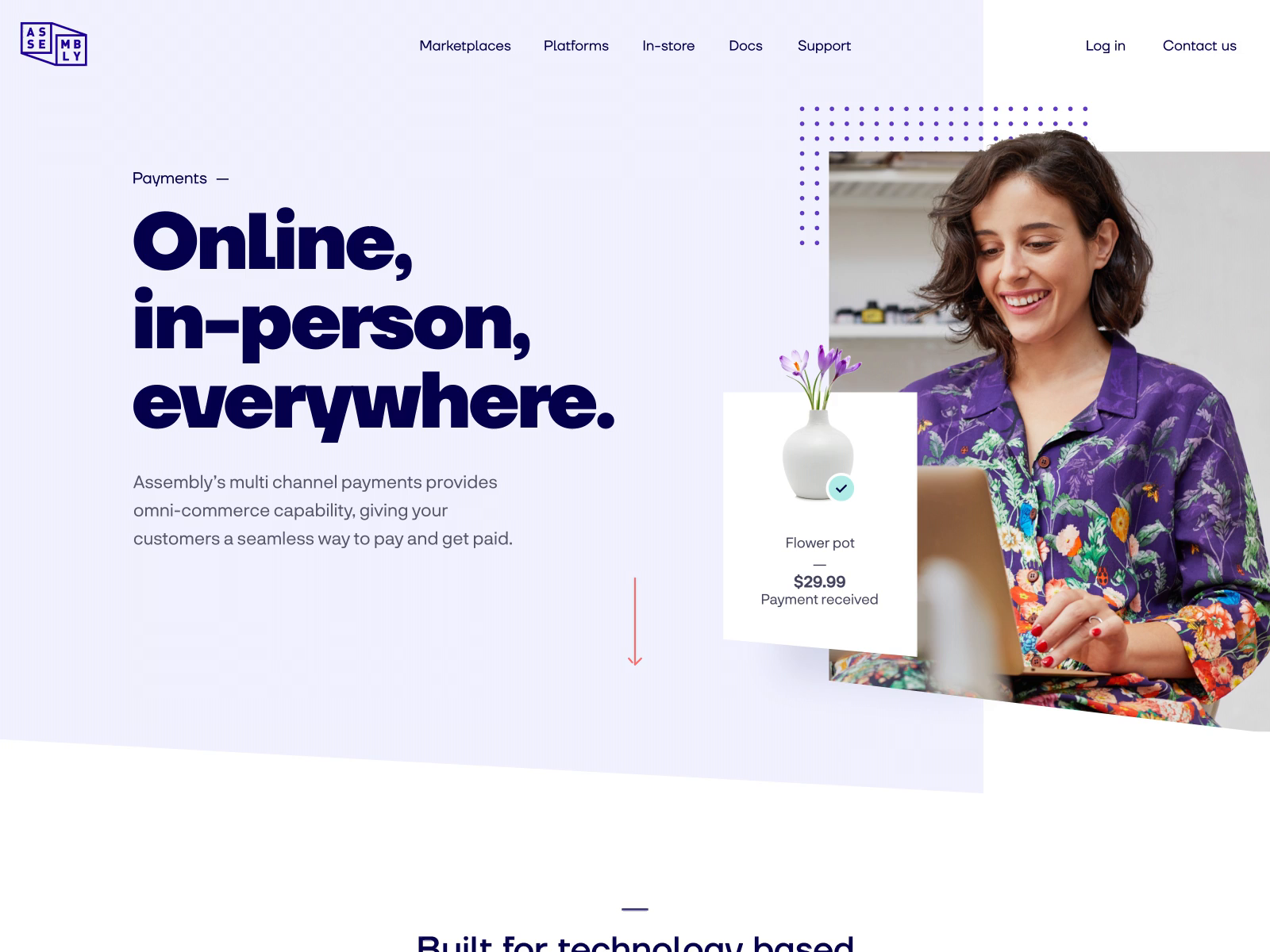Screenshot of Assembly Webpage:

The image is a screenshot of a webpage for the platform "Assembly." The page has a distinct rectangular shape, suggesting it is not a phone screenshot. In the top left corner, the Assembly logo is prominently displayed, featuring two interlocking squares. The top middle section of the page contains a navigation bar with the headings: Marketplace, Platform, In-Store, Docs, Support. On the top right, there are links for "Login" and "Contact Us."

The background of the webpage transitions from white to light purple, separated by a series of small dots. Centered prominently in the main section is an image of a Caucasian woman with short hair, wearing a colorful shirt in green, red, and purple hues. She is smiling while looking at her computer.

Next to the woman, there's an image of a flowerpot containing a few purple flowers. A checkmark icon indicates that a payment has been received for the item, which is listed as "Flowerpot" at a price of $29.99.

On the left side of the webpage, there is a section heading titled "Online, In-Person, Everywhere," under which there is a descriptive subtitle: "Assembly's multi-channel payment provides omnicommerce capability, giving your customers a seamless way to pay and get paid." Positioned in the middle of the screen, to the right of this text, is a downward-facing vertical red arrow, drawing attention to additional content below.

Overall, the page highlights the platform's capabilities in providing diverse payment methods and a seamless transaction experience for users.